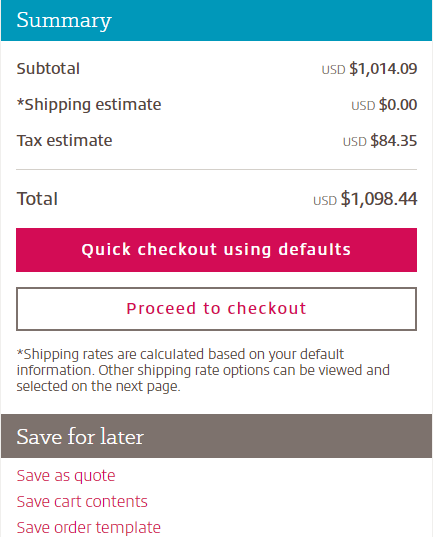The image is a screen capture of an order summary interface. At the top of the image, there is a blueish-teal border with the text "Order Summary" prominently displayed. Below this title, the detailed costs are listed in brown text, starting with "Subtotal" at USD $1,014.09. Following the subtotal, the "Shipping Estimate" is indicated as USD $0, with a small asterisk next to it. The "Tax Estimate" is listed as USD $84.35. Finally, the "Total" amount is USD $1,098.44.

Just below these figures, there is a pink box with white text that reads "Quick Checkout Using Defaults." This box appears to be selected. Beneath it, a white box with pink font and a gray border contains the text "Proceed to Checkout."

Further down, a message in gray text, accompanied by an asterisk, explains, "Shipping rates are calculated based on your default information. Other shipping rate options can be viewed and selected on the next page."

At the bottom, there is a gray box with white text that says "Save for Later." Following this, several options in pink font are listed: "Save as Quote," "Save Cart Contents," and "Save Order Templates."

The text throughout the image is very clearly worded, large, and easy to read, with no pixelation or blurring, making it extremely user-friendly and straightforward.